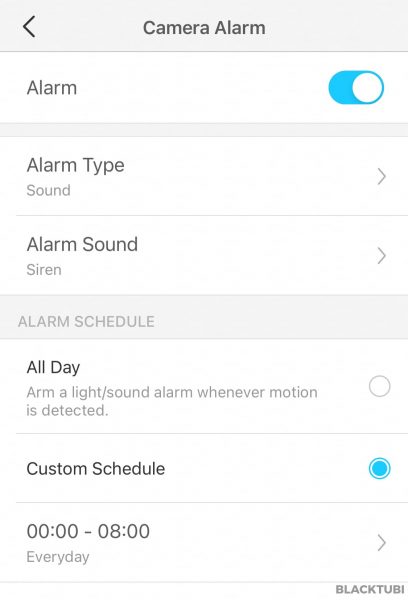A mobile phone screenshot displays a camera alarm settings interface. The background is white, with black text for easy readability. At the top, there is a gray header bar labeled "Camera Alarm" with a back button and arrow in the upper left corner. Below that, the interface indicates that the alarm is turned on, with a blue slider button signaling its active status; it likely turns gray when off. The "Alarm Type" is specified as "Sound" and the "Alarm Sound" is set to "Siren," suggesting it would emit a loud, disturbing noise. Further down, another gray header reads "Alarm Schedule." Here, the user can select between "All Day" or a "Custom Schedule." The custom schedule option has been selected, with settings configured for "Every Day" from "0000 to 0800," indicating the alarm will be active throughout the night.